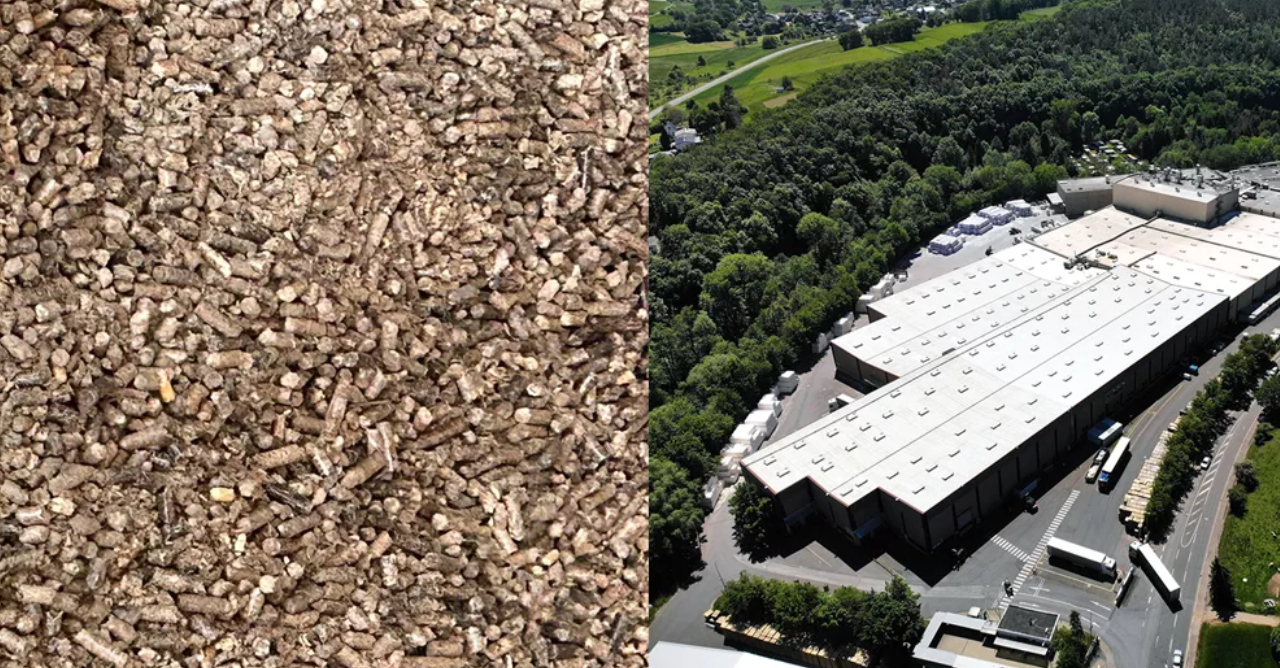The image is comprised of two photographs side-by-side. The left photograph depicts a close-up view of a large pile of wood pellets, scattered and varying in color from brownish to lighter shades. These pellet-shaped objects occupy the entire frame, creating a textured surface.

The right photograph is an aerial view of a large warehouse complex with multiple connected sections, spanning diagonally from the middle upper portion to the lower left corner of the image. The building appears to be one or two stories high with a flat, whitish roof. Around the warehouse, there is a parking lot populated by at least four tractor-trailer trucks in various positions. Smaller trucks are also parked, suggesting a busy logistical hub. The right side of the picture is bordered by a dense area of green trees, indicating a wooded region, with a grassy area visible in the background.